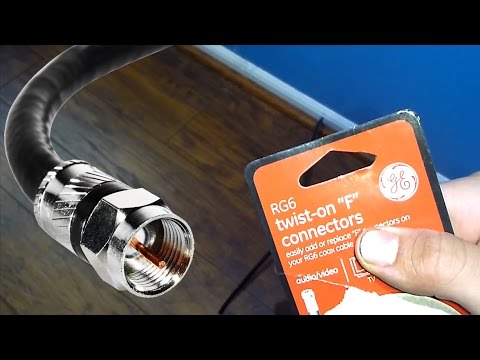The image depicts a close-up of a General Electric (GE) coaxial cable, prominently featuring an RG-6 twist-on F connector. On the left side of the image, a thick black cable is visible, capped with a silver metal end exposing a central copper conductor and surrounding shielding. The foreground showcases a light-skinned hand holding up an orange card with white font and a black border, detailing the product's specifications: "GE RG-6 twist-on F connectors. Easily add or replace F-connectors on your RG-6 coax cable." This packaging indicates its use for enhancing audio and video signal quality by preventing interference. The background consists of dark brown hardwood flooring at the bottom and a dark blue painted wall on the right. The image captures the essence of the coaxial cable's purpose and its practical presentation.